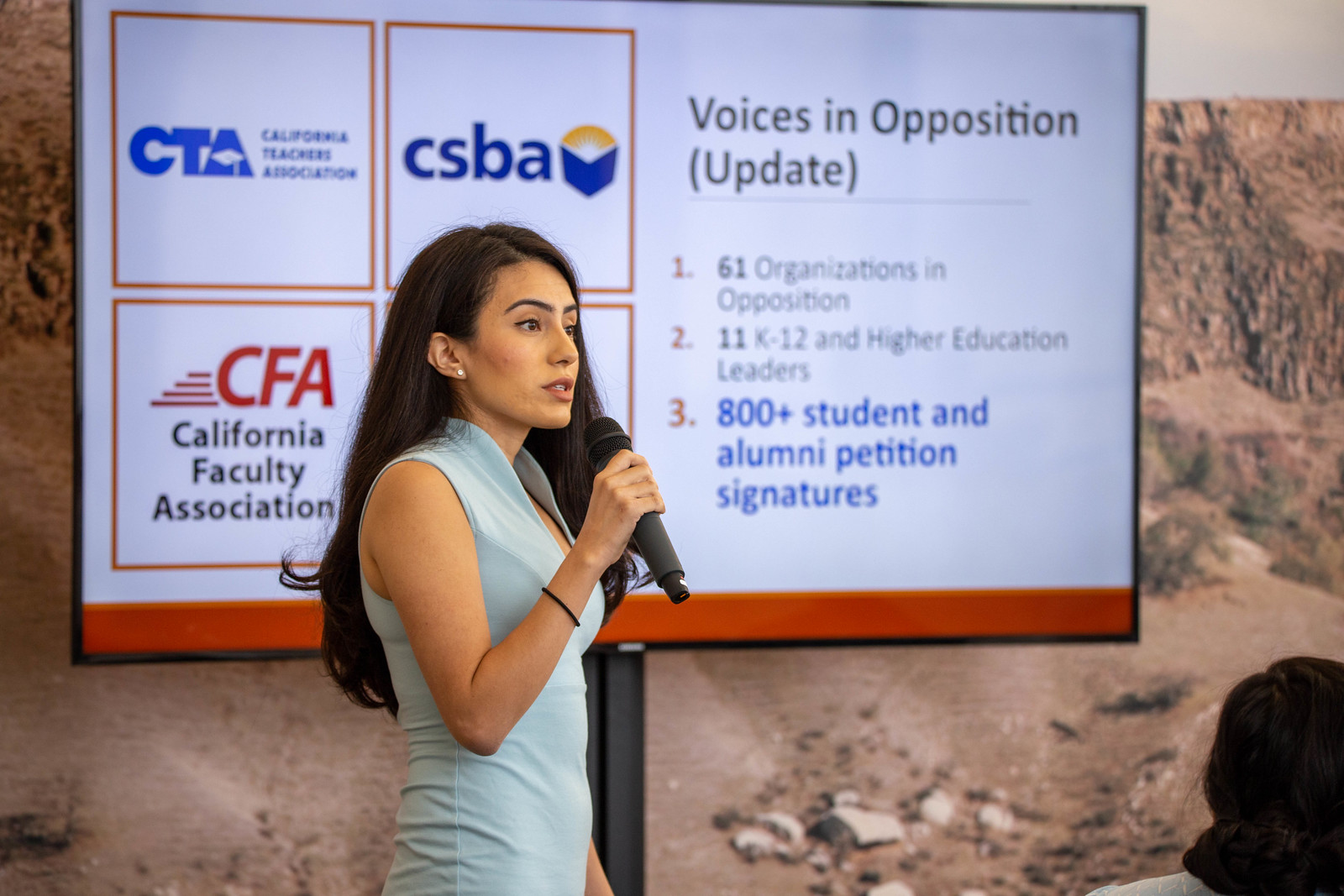In the image, a professionally presentable woman is giving a presentation. Standing in front of a large screen monitor, she has dark brown hair that reaches the center of her back and brown skin. She is dressed in a sleek, form-fitting blue dress with a popped-up collar and is wearing little diamond stud earrings along with a black bracelet on her wrist. Holding a black microphone up to her partly open mouth, she appears to be speaking, her eyebrows raised and her gaze directed towards the right side of the screen.

Displayed on the large screen behind her is a slide titled "Voices in Opposition Update," which lists three bullet points: "1. 61 organizations in opposition," "2. 11 K-12 and higher education leaders," and "3. 800+ student and alumni petition signatures" in blue, bold text. The slide features a white background with an orange bar running across the bottom. On the left side, there is a grid of logos for four organizations. The visible ones include the California Teachers Association (CTA) in the top left, a logo with a blue book and yellow arch labeled CSBA in the top right, and the California Faculty Association (CFA) in the bottom left. The fourth logo is obscured by the woman herself.

Additionally, a partial view of another person can be seen in the bottom right corner of the image, with only the back of their head visible. The wall behind the slide appears to have an artwork depicting a desert.